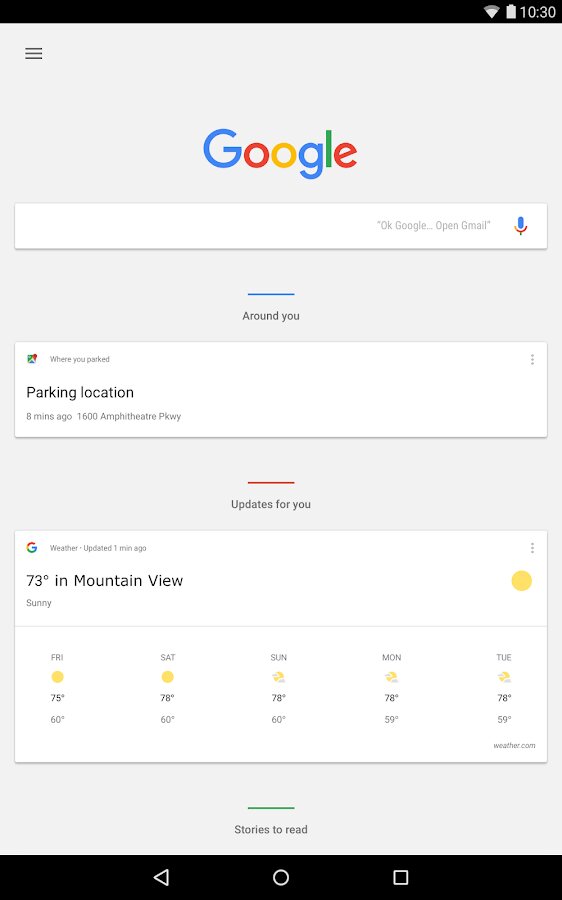The image showcases a smartphone displaying the "Googly" homepage with meticulously detailed elements. At the top left of the screen, the current time is visible, while the top right corner displays the date, a battery icon, and a Wi-Fi signal icon. The centerpiece of the screen is the "Googly" logo, vibrantly colored: the first 'G' in blue, the first 'O' in red, the second 'O' in yellow, the second 'G' in blue, the 'L' in green, and the 'E' in red.

Beneath the logo, a search bar reads "Ok Googly, open Gmail," indicating a voice recognition prompt. Below, it lists suggestions and relevant updates like "around you" and "where you parked," detailing a parking location 8 minutes ago at 1600 Amphitheatre Parkway.

The lower section provides updates including a dynamic weather report, noted as updated one minute ago, indicating it's currently sunny and 73 degrees in Mountain View. A forecast is displayed, mapping out the weather from Friday to Tuesday: 
- Friday: 75 degrees, low of 60
- Saturday: 78 degrees, low of 60
- Sunday: 78 degrees, low of 60
- Monday: 78 degrees, low of 59
- Tuesday: 78 degrees, low of 59

Further down, a "Stories to Read" section appears, providing curated news articles. Finally, at the very bottom, familiar smartphone navigation buttons are present: Back, Minimize, and Reset. This detailed caption captures the immersive experience offered by the Googly homepage on a smartphone screen.